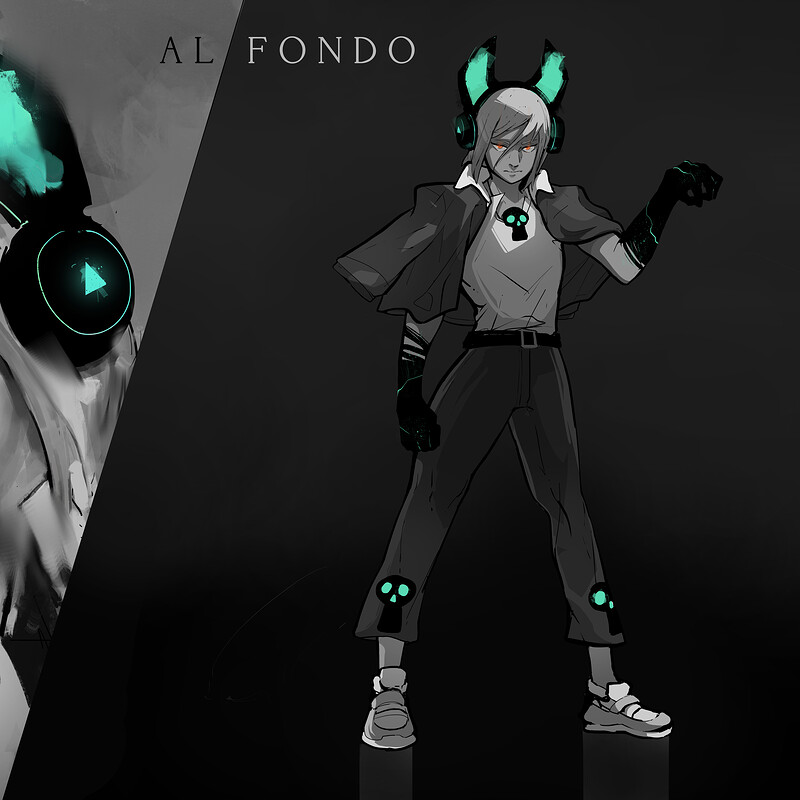The image depicts a character named Alphondo, showcased in an anime-inspired black and white illustration with vibrant green accents. Alphondo wears elaborate headphones resembling ears, featuring a cyan inside that appears to glow, giving an almost fiery effect. The character has medium-length hair and a distinctive green necklace adorned with a black skull that has green eyes. Alphondo sports a coat draped over his shoulders, revealing a grayish-white dress shirt underneath, paired with black gloves, a belt, and gray pants that end with skull motifs mirroring the one on the necklace. The image composition includes a unique setup with the character's right hand extended against a dark gray backdrop, while the left side highlights a close-up of the cyan headphones. The word "Alphondo" is split stylistically across the top, with "AL" on the left gray side and "FONDO" on the right darker side. Alphondo's footwear consists of sports shoes, and there's a visible reflection of them at the bottom of the picture.